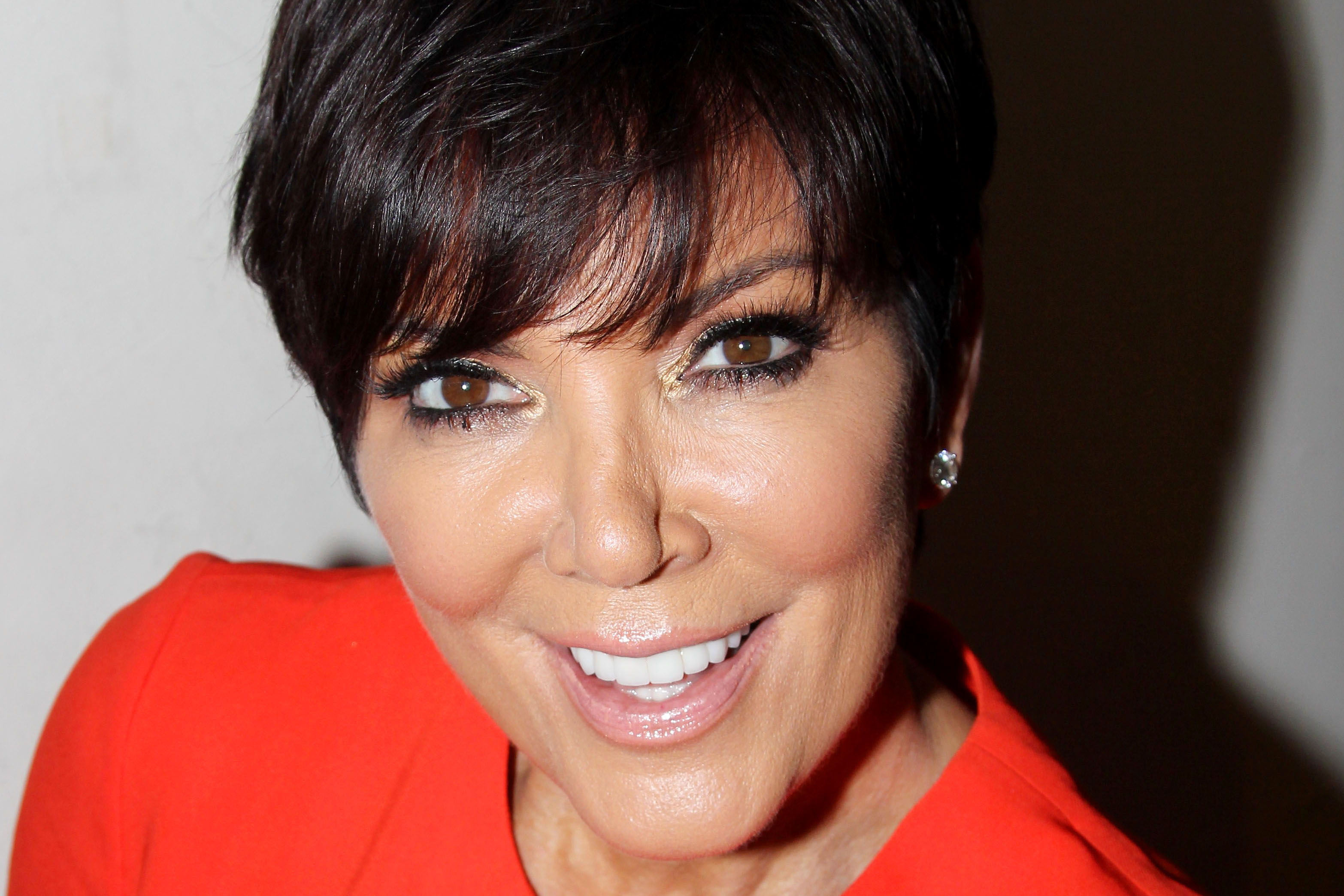The image is a professional promotional photograph of Kris Jenner from the Kardashian family. She is facing forward, with her profile captured from her upper shoulders to just above her eyes, though the top of her head is slightly cut off by the photograph's edges. Kris is smiling warmly, showcasing a bright, confident smile that partially reveals her lower teeth and fully reveals her upper teeth. Her short, black, wispy pixie hair is brushed slightly to the side.

Kris is adorned with shimmery, diamond-studded earrings, and she is wearing a striking orange-red top. The shot is highly focused and well-lit, enhancing the colors and details of her appearance. Her eyes, brown and detailed with black eyeliner and substantial eye makeup, are looking directly into the camera, creating a direct and engaging connection with the viewer.

The background is a plain, light gray with Kris's shadow clearly visible behind her, adding depth to the shot. The entire setup, combined with Kris's poised expression, suggests a deliberately contrived and polished promotional photograph.